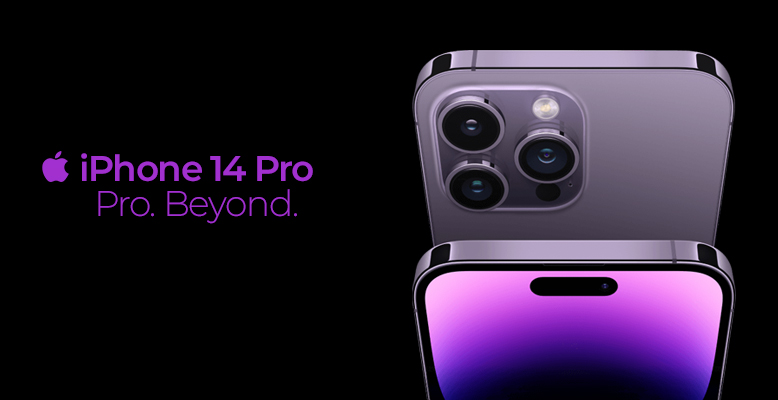This advertisement features a sleek, minimalist design on a black background within a horizontal rectangular frame. On the left, a vivid purple Apple logo with a rounded bite taken out of its top right corner draws immediate attention. To its right, bold purple text reads "iPhone 14 Pro," while a thinner line of text underneath proclaims "Pro Beyond" in the same striking purple hue.

To the right side of the text, there are two overlaid images of the iPhone 14 Pro. The top image showcases the phone's back, angled to highlight its design. It features a square section with rounded corners in the top left, housing three lenses. The top-left lens is encircled by a thick black outline and contains a small, luminous blue center. Below it, a second lens with a slightly thinner black outline and a similarly sized, perhaps slightly larger, blue center is aligned directly below. Centered between these two lenses on the right is a third lens with a larger, gleaming blue center and a thin black outline. Above this central lens, a metallic-looking small circle reminiscent of a CD adds an intriguing detail, with a simple black circle situated beneath it. The phone’s outline is metallic and reflective, exuding a sense of premium quality.

In front of this top image, slightly lower and just beneath the square lens array, is another view of the phone showcasing its front side. The screen displays a captivating purple gradient that transitions from pink at the top to black at the bottom, with various shades of purple blending seamlessly in between. This careful layering and detailing emphasize the phone's sophisticated design and advanced features, perfectly aligning with the "Pro Beyond" slogan.